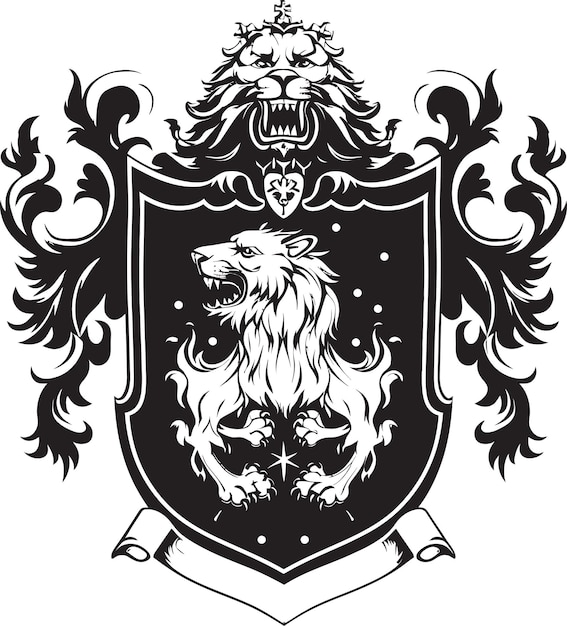The image depicts a detailed black-and-white coat of arms or family crest set against a white background, seemingly created digitally. At the top of the crest, a lion with a snarling expression and a crown shaped like a mini cross on its head peers over a black shield. The lion’s head rests atop the shield, which features a secondary lion within its confines. This second lion, rendered in white with black accents, is positioned in a heraldic stance with contorted legs and all paws facing inward, its body angled to the left and mouth agape in a growl. Surrounding the shield, black filigree elements or flame-like details extend outward from either side. Below the shield, there is a matching white ribbon banner with no inscription, framed by a black outline. The intricate design includes decorative scrolls and a pattern of little white circles and stars amid the filigree, adding to the complexity and artistry of the emblem.